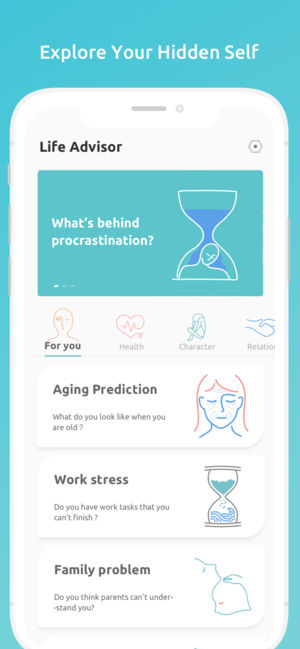In this detailed screenshot of a LifeAdvisor webpage viewed on a smartphone, the interface is predominantly blue, with key text sections in white. At the top, an inspirational tagline invites users to "Explore Your Hidden Self," suggesting personalized self-discovery tools available on the site. Prominently displayed is the LifeAdvisor logo, followed by a feature section titled "What's Behind Procrastination," accompanied by an illustrative image of an hourglass symbolizing the passage of time.

Below this are several clickable areas for users to delve into specific life aspects: the highlighted "For You" section, "Aging Prediction" featuring a sketched image of a girl, "Work Stress," and "Family Problems." Each of these sections implies tailored advice or assessments to help users understand various facets of their lives, thus enhancing their self-awareness and personal development journey.